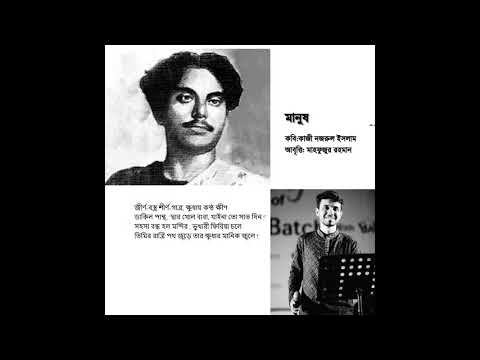In the center of this black-bordered, black-and-white photograph, there are four distinct sections arranged in a square grid. The top left quadrant features a close-up of an Arab man with short black hair and a mustache, wearing a black and white t-shirt, gazing thoughtfully into the distance. The top right and bottom left quadrants contain blocks of black foreign text, possibly Arabic, on a white background. The bottom right quadrant shows another man standing confidently in front of a podium, dressed smartly, smiling, and seemingly giving a speech. Each section's components starkly contrast in their composition, adding depth and a narrative feeling to the overall image.